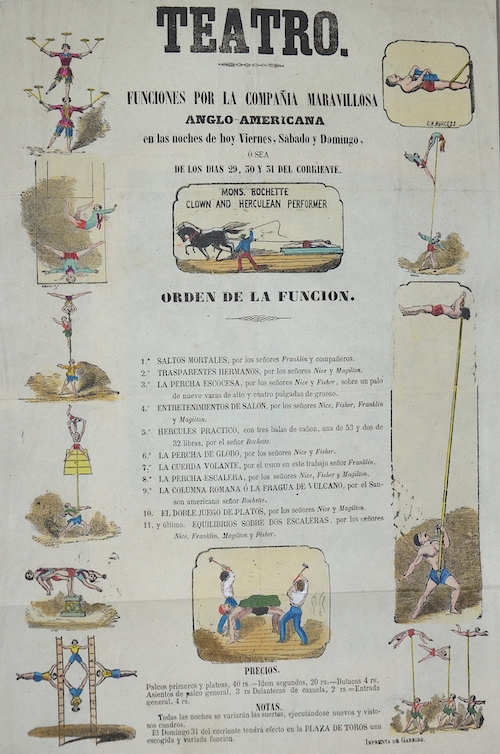The image is of a vintage Spanish poster titled "Teatro" in bold black text at the top, likely referring to a theater or performance event. The poster, which appears to be around 30 to 40 years old, features detailed, colored illustrations of various circus acts arranged vertically on both the left and right sides. These acts include a person spinning dishes, trapeze artists, acrobats balancing on each other, and performers with a long pole. There are people depicted wearing blue pants and a black horse included in the illustrations. Additional text on the poster reads, "Funciones por la Campaña Marveloso Anglo-America en las noches de hoy, viernes, sábado y domingo," indicating shows happening on today's date, Friday, Saturday, and Sunday. The poster also lists "Orden de la Funcion," suggesting a sequence of performances. The overall effect is a detailed instructional or promotional diagram for a series of circus-themed events.